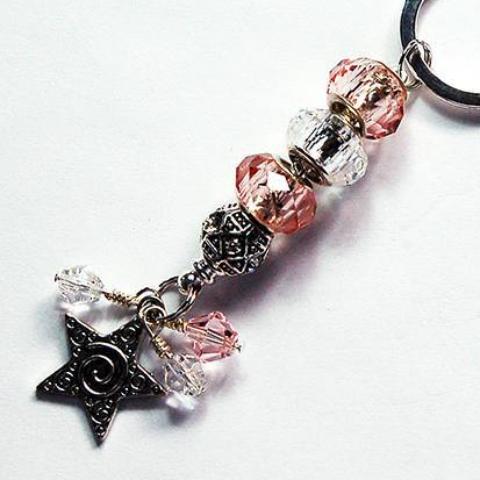This close-up, colored photograph showcases a detailed charm or piece of jewelry arranged diagonally with a white background. The bottom left of the image features a flat, silver star with a spiral engraving in the middle. Moving upwards diagonally towards the top right, the charm is composed of a series of circular beads, beginning with a black bead adorned with intricate designs, followed by a pink bead, a clear bead, and another pink bead. These beads are connected via a small silver loop to a thread or chain, which is hinted at in the top half of the image. The entire charm appears to be attached to a silver hook or ring, suggesting it could be part of a keychain or necklace. This intricate piece of jewelry prominently fills the frame, emphasizing its detailed craftsmanship and vibrant colors.